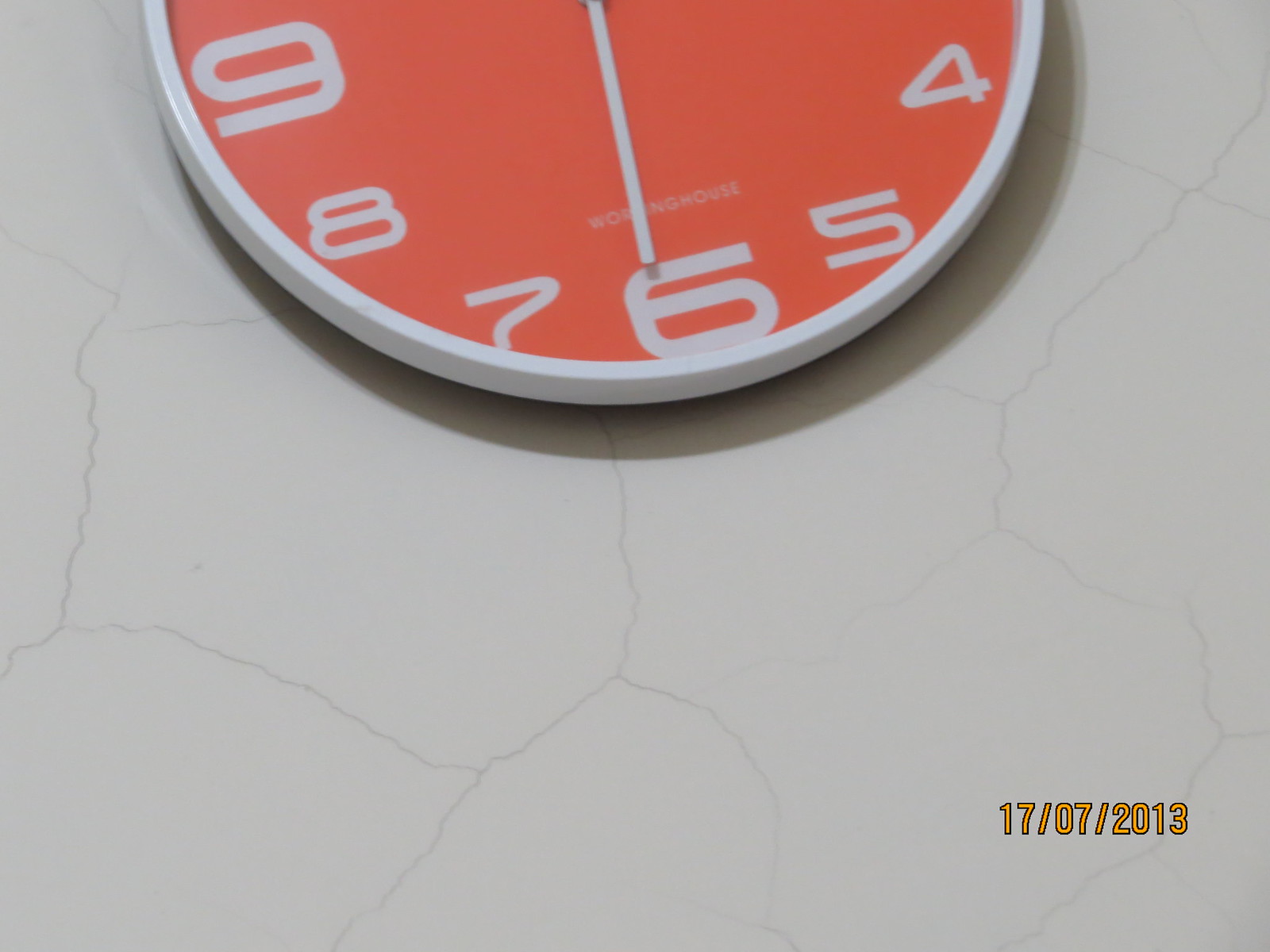This image captures the lower half of a round clock, prominently showcasing the numbers 4 through 9 in white against an orange background. The clock's quarter hour numbers, particularly 6 and 9, are markedly larger than the intervening ones. The big hand indicates 6, suggesting the time might be around half past an hour. Below the clock face, the words "WORKING HOUSE" are visible. The clock appears to be either resting upon or mounted against a light gray surface with noticeable surface cracks. Additionally, the bottom right corner of the square-shaped image displays the date "DAY 17, MONTH 7, YEAR 2013," corresponding to July 17, 2013.